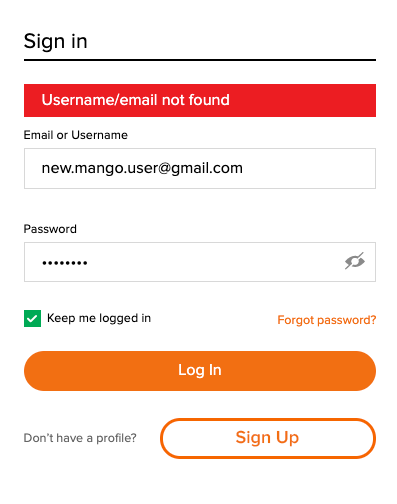The image depicts a sign-in screen on a smartphone. At the top of the screen, bold text reads "Sign In," with a solid black line beneath it. Below this, a prominent red alert rectangle displays a white error message: "Username/Email not found." The screen includes an entry field labeled "Email or Username," into which a user has typed "new.mango.user@gmail.com." 

Below the username field, there is a password field featuring approximately eight concealed characters, indicated by black dots. To the right of the password field is an eye icon with a slash through it, signifying that the password is hidden. 

Further down, a green checkbox, marked with a white checkmark, is labeled "Keep me logged in." Adjacent to this checkbox is a "Forgot Password?" text link. 

At the bottom of the screen, there is a large, orange capsule-shaped button that spans almost the entire width of the screen. This button displays the text "Log In" in white. Beneath this button, on the left side, gray text asks, "Don't have a profile?" To the right, there is a white capsule-shaped button with an orange border and orange text that reads "Sign Up." This sign-up button is notably narrower than the login button above it.